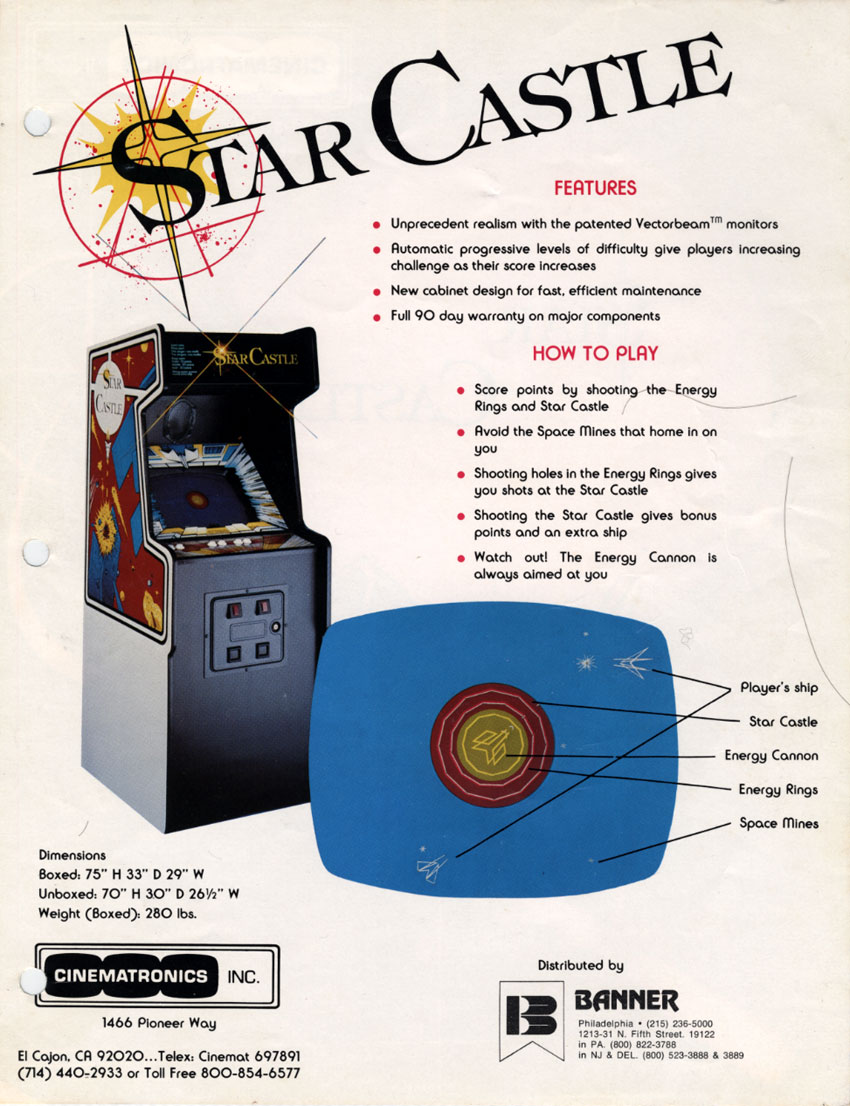This is an image of an old-school advertisement for the 1980s arcade video game machine called "Star Castle." At the top, large blue letters spell out "Star Castle," with a distinctive logo featuring a red circle, black star, yellow sunburst, and red splatter overlaying part of the text. This ad is richly detailed and entirely graphic, devoid of actual photographs but possibly including computer-generated imagery or artwork.

To the right of the logo, the ad lists "Features" in red text, followed by red bullet points detailing the impressive qualities of the machine: unprecedented realism with patented vector beam monitors, automated progressive difficulty levels, new cabinet design for fast maintenance, and a 90-day warranty on major components. Below this section, another heading in red text reads "How to Play," with black text instructions and red bullet points explaining the gameplay: players score points by shooting energy rings, avoid homing space mines, and aim for the star castle to earn bonus points and extra ships while dodging an ever-aiming energy cannon.

The bottom section of the advertisement showcases a representation of the game screen, featuring a central bullseye with a spaceship silhouette and arrows identifying key elements such as Player Ships, Star Castle, Energy Cannon, Energy Rings, and Space Mines. Alongside this graphic, there is a depiction of the actual gaming machine.

On the lower part of the ad, it provides the physical dimensions of the game machine—75 inches high, 33 inches deep, and 29 inches wide when boxed, and slightly smaller when unboxed. The machine weighs 280 pounds. Also included is the contact information for the manufacturer and distributors: Cinematronics Inc., with an address at 1466 Pioneer Way, El Cajon, California, 92020, and phone numbers 714-440-2933 and toll-free 800-854-6577. Additionally, the distributor information for Banner in Philadelphia, New Jersey, and Delaware is provided along with their respective contact details. The ad exudes a nostalgic, vintage feel, reminiscent of the classic flyer style seen in the heyday of arcade gaming.